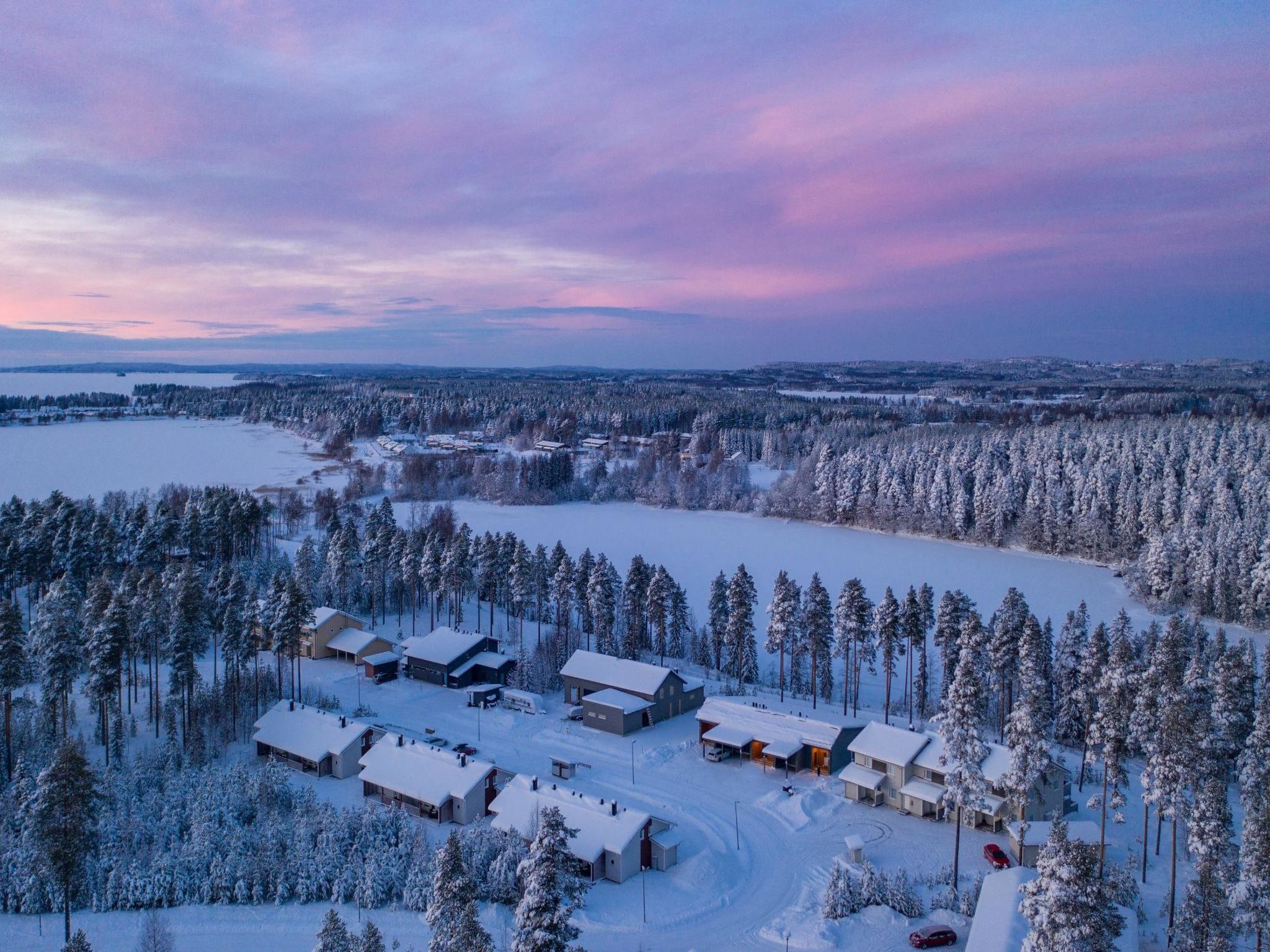An aerial photograph captures a serene, snowy landscape under a dawn or dusk sky, where the horizon glows in shades of blue and purple interspersed with white and gray clouds. The foreground is dominated by snow-clad roofs of small, industrial buildings, potentially serving as garages, brown and gray in color. In the middle ground, three such buildings are part of the snowy scene, while a row of approximately six structures lines the background towards the right. No people are visible. The left side and background showcase a picturesque view of pine trees, their branches heavy with snow, encircling the buildings. Amid this winter wonderland, bodies of water, partially frozen and snow-capped, punctuate the scenery on the left and middle-right portions, while the entire ground is blanketed in pristine white snow.